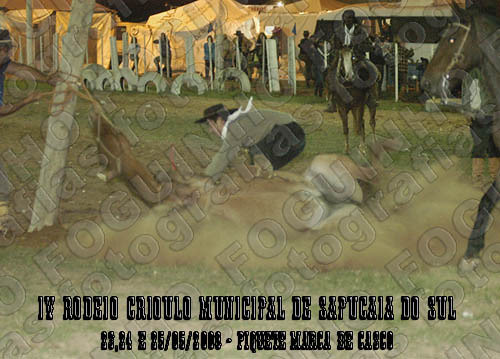This image portrays a dynamic scene with a cowboy theme, possibly at a rodeo or rural gathering. Central to the image is a person clad in a black cowboy hat, a gray shirt, black pants, and a white bandana kneeling on the ground. This cowboy appears to be handling or perhaps being thrown off a horse, which is surrounded by a plume of dust suggesting movement and action. The horse, with a saddle wrapped around it, has its head and feet visible on the right side of the photo, emphasizing the chaos of the moment.

In the background, another individual dressed in dark attire and a white bandana is riding a horse, adding depth to the scene. The setting is a grassy field with white-painted half-tires embedded in the ground, functioning as makeshift fencing. Further adding to the visual complexity, there are people behind these barriers, possibly audiences, suggesting that this might be an event area.

This photograph has a transparent watermark with the text "Foguinho Fotografias" diagonally across it, indicating the photographer's branding. Additionally, the image is overlaid with text in old saloon-style Spanish font at the bottom, offering some municipal information and a date, albeit hard to discern due to its small size and the photo’s overall low resolution and slight blur. This adds a historical or rustic charm to the image, making it resemble an antiquated photograph despite its indistinct details.